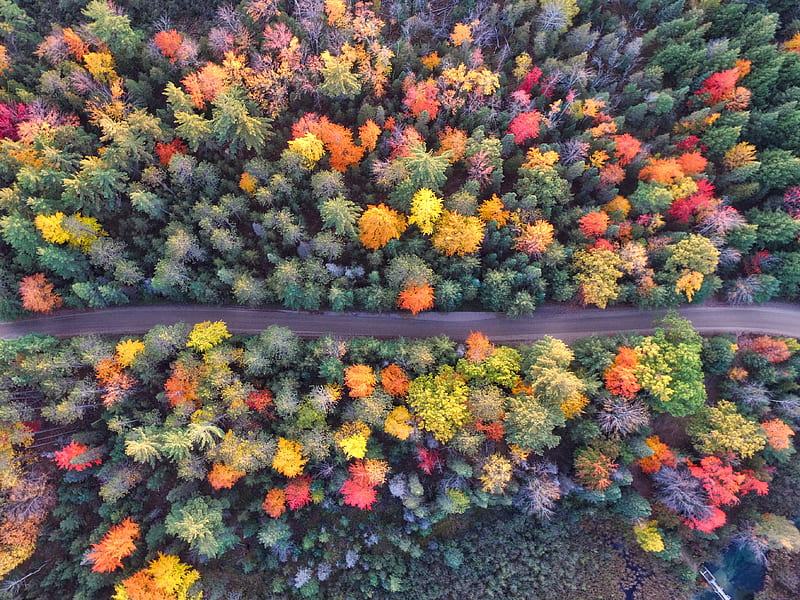This is a large square aerial view looking straight down at a winding, two-lane road that stretches horizontally from left to right through the center of a dense forest in early fall. The vibrant foliage creates a spectacular array of colors ranging from greens and yellows to oranges, reds, magentas, and even blues and purples, painting a vivid landscape. The tops of the trees are packed closely together, enveloping the road entirely on both sides. The forest extends across most of the image, but as you move towards the bottom right corner, it gives way to a marshy area with sparse, low-lying foliage and visible water bodies, suggesting a wetland. A small bridge may be present over one of these water patches, adding a touch of human engineering to the natural beauty. The road itself is devoid of any vehicles, enhancing the serene and undisturbed atmosphere. The image captures the enchanting beauty and tranquility of the scene, highlighting the diversity of the fall colors and the harmonious blend of nature and the solitary road cutting through it.